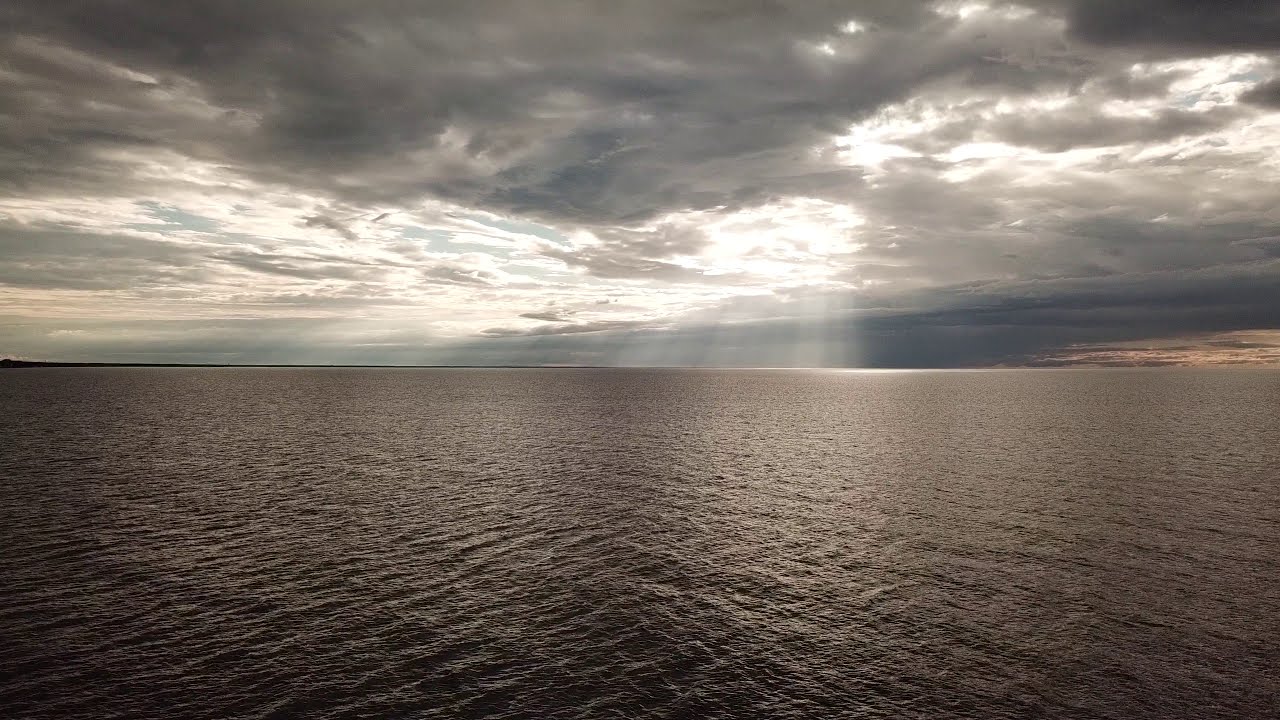An aerial photograph captures a vast, tranquil body of water, likely the ocean or a large lake, with the predominant hues being gray and brown. The water's surface is rippled, reflecting the minimal sunlight that pierces through the thick, overcast sky. Dark gray and black clouds dominate the sky, with a few openings allowing sun rays to stream down in striking, almost ethereal beams that illuminate sections of the water. The horizon is largely empty, devoid of houses or trees, lending an expansive, open feel to the image. Along the left edge of the horizon, a thin black land mass extends partially into the frame before fading out. The daylight in the image is subdued, contributing to an overall somber and atmospheric mood. Some parts of the sky near the horizon glimmer with hints of orange, suggesting it could be evening. Brown, barren hills line the distant shore, completing the desolate but captivating scene.